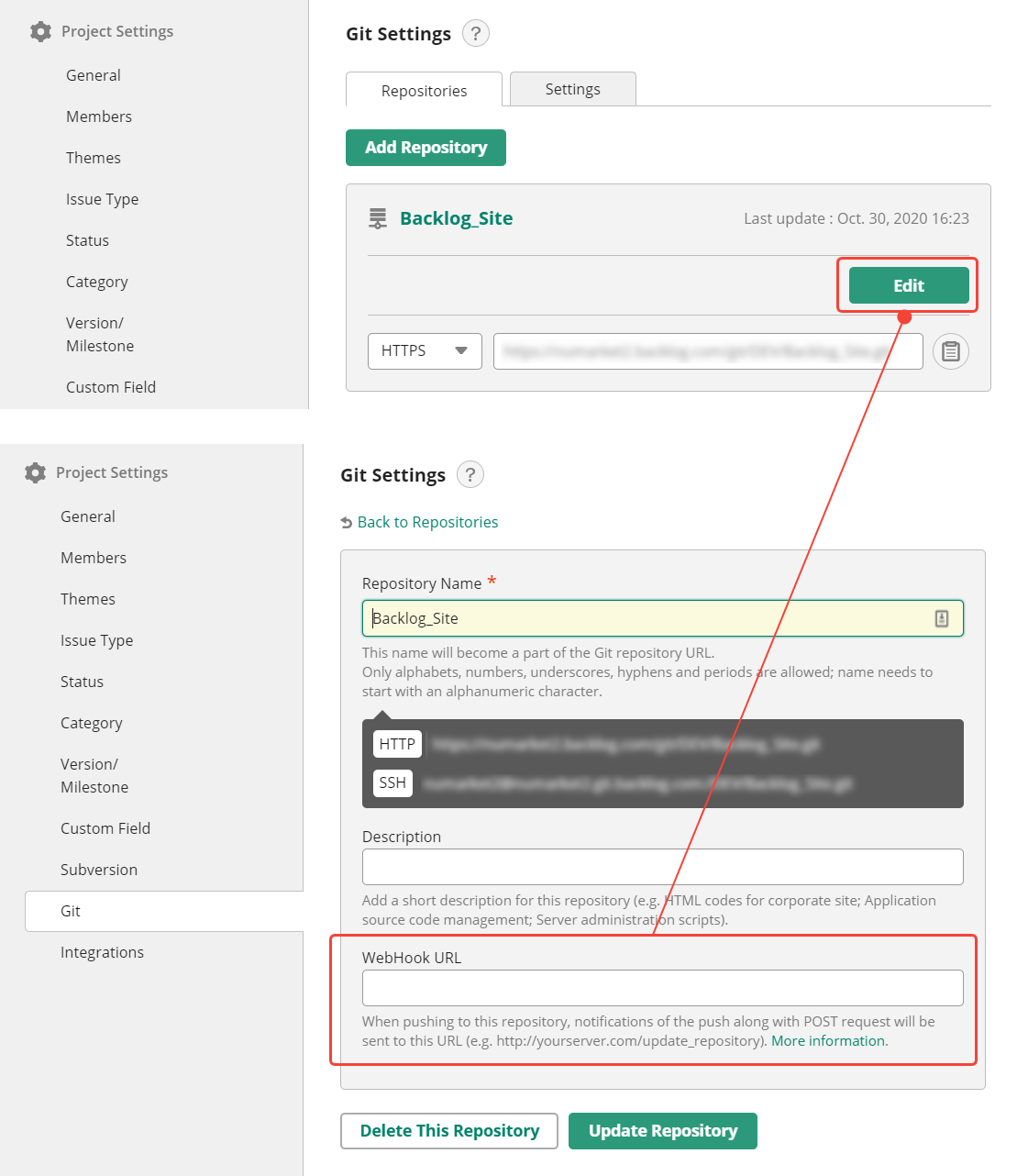A detailed screenshot from a tablet displays the user interface of a GitHub-related website, featuring sections dedicated to project management and repository settings. The interface is set against a minimalistic white background, with pale blue highlighted boxes positioned along the upper left and left side of the screen, including options such as Project Settings, General, Members, Themes, Issue Type, Status, Category, Version, Milestone, Custom Field.

Situated to the right is a prominent, bolded heading labeled "Get Settings," accompanied by an informational question mark icon and an active tab titled "Repositories." Beneath this setup is a noticeable green button with white text reading "Add Repository." Below the button, there is a pale blue box displaying the text "Backlog_Site" in green, coupled with an Edit button also highlighted.

At the bottom of the interface, a specific section outlined with a red border catches the eye. This section is connected by a line to another box further down the page and takes up the right two-thirds of the screen. It is labeled "Webhook URL," explaining that when pushing to the repository, notifications along with a post request will be sent to this URL. The screen is prompting for the addition or editing of a Webhook URL and includes partially obscured options for HTTP and SSH, likely for configuring secure connections.

Overall, the screen captures detailed functionalities for managing and customizing GitHub repositories through a clear and organized layout.